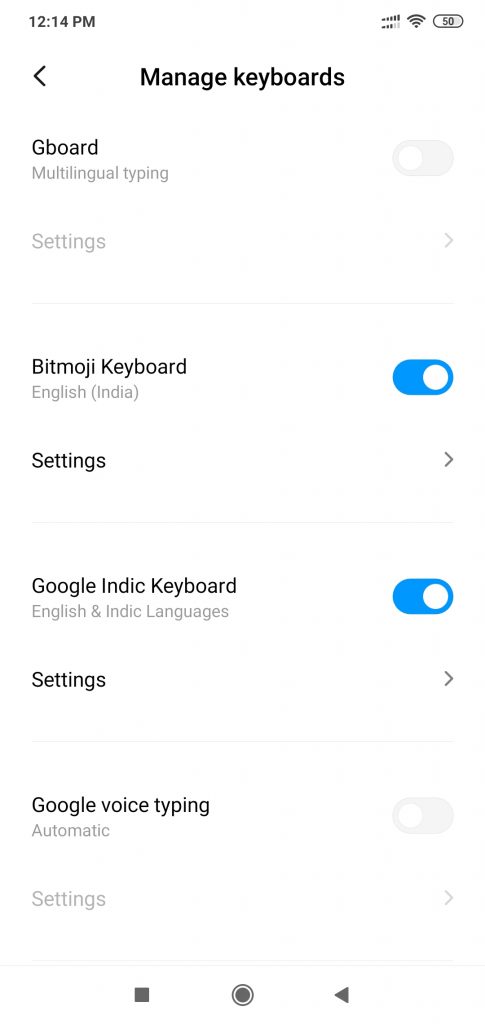A screenshot of a smartphone display shows the following details:

- At the top-left corner, the time reads 12:14 PM. Icons for Wi-Fi, network signal strength, and battery status are also visible.
- Below the status bar, there is a "< Manage keyboards" header.
- The first entry is labeled "Gboard - multilingual typing" with a toggle switch beside it in the "off" position. "Settings >" is displayed to its right, and a light gray horizontal divider line follows beneath it.
- The second entry reads "Bitmoji Keyboard (English and India)" with an active blue toggle switch beside it. To its right, it says "Settings >".
- The third entry shows "Google Indic Keyboard (English and Indic languages)" with another active blue toggle switch. The "Settings >" option is also visible here.
- Following another light gray divider line, the final entry is "Google Voice Typing (automatic)" with the toggle switch in the "off" position. The "Settings >" option is shown here as well.